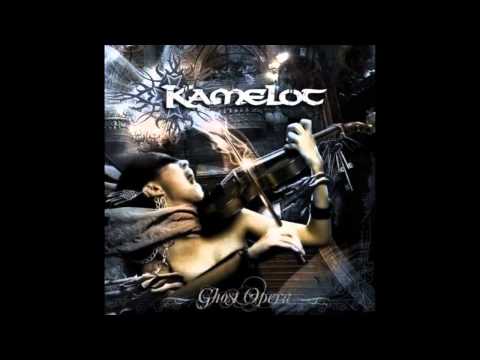This rectangular image, framed by a large black border—thinner on the top and bottom, and wider on the sides—appears to be an album cover. The central portion is a bustling, dynamic scene. The top of the image features the word "Camelot" in white letters with streaks of black running through them, stylized as K-A-M-E-L-O-T. Below this title, in thin white cursive script, are the words "Ghost Opera."

In the heart of this composition stands a person intensely engaged in playing a violin. Details such as black coverings over their eyes and head, and chains hanging from their right earlobe, add to their enigmatic appearance. They firmly grasp the violin with their left hand, while the right hand wields the bow, accentuating their fervor for the music. The violin itself is a dark brown, accentuating the overall somber theme. Surrounding this musician is a surreal, chaotic background that includes lightning strikes, stone stairs ascending to what seems like a castle, and what might be considered tentacles wrapping ominously around the person’s throat and arm—hinting at an eerie, almost monstrous presence.

The dark, intense backdrop is accentuated with colors primarily in shades of black, with occasional bursts of purple and blue. The entire scene conveys a sense of dramatic tension and gothic beauty, fitting the evocative title "Ghost Opera." The elements collectively suggest this is an album cover, likely designed to invoke a sense of dark fantasy or operatic grandeur.